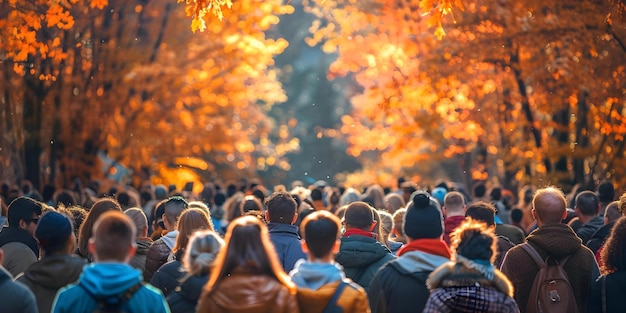The photograph captures a vibrant outdoor scene on a bright autumn day. The composition features a substantial crowd forming a large throng that extends from the foreground into the distance. The people, varied in age and gender, are walking along a central pathway and are dressed in warm, winter or fall-themed attire, including knit hats, sweaters, jackets, and coats, indicating the season is fall. On both sides of this pathway, the image is framed by trees adorned with an array of autumn leaves, ranging in color from dark to light orange and yellow. The trees appear to be arching slightly, creating a tunnel-like effect over the crowd. Natural light, seemingly originating from the center of the image, illuminates the scene and creates a poetic ambiance as it reflects off the individuals' heads. The precise reason for the crowd's forward focus remains unclear, adding an element of intrigue to the picturesque and serene setting.